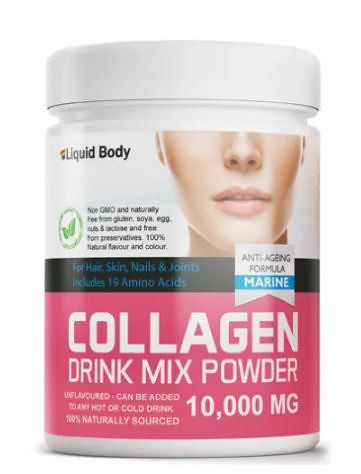This image displays a cylindrical white container with a matching white lid. A label is affixed to its body, prominently featuring the bottom half of a woman's face with fair, somewhat brownish skin. On the top left of the label, the black text "Liquid Body" is displayed, accompanied by a green leaf symbol denoting non-GMO and natural status, and claims such as "free from gluten, soy, egg, nut, and lactose, and free from preservatives." Additional smaller text indicates it offers 100% natural flavors and color, beneficial for hair, skin, nails, and joints. Toward the bottom, a conspicuous pink band features the text "Collagen Drink Mix Powder 10,000 mg" in white letters, with a black band above it that includes an "anti-aging formula" banner and the term "marine." This overall presentation suggests the product is a health-focused collagen supplement.